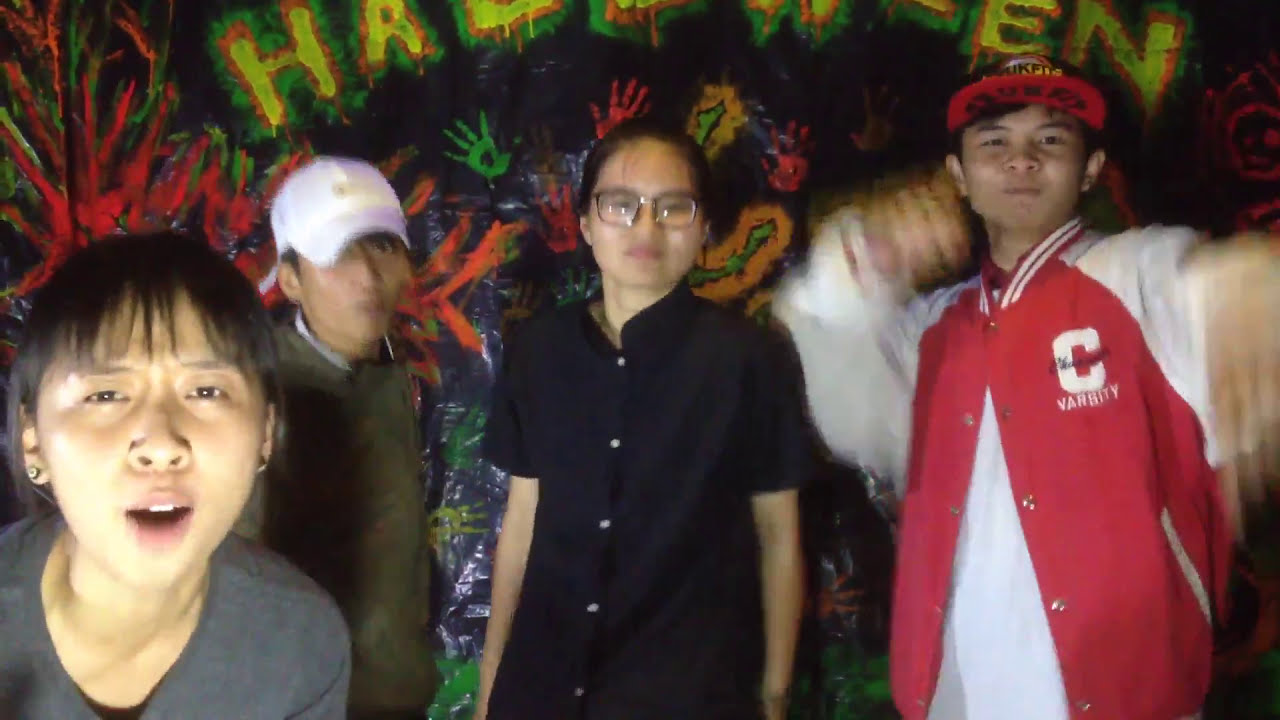In this lively image, four Asian youths, possibly in their late teens or early twenties, are gathered in front of a vibrant mural that features the word "Halloween" in a mix of green, orange, red, and black colors, along with various handprints. Each individual engages with the camera in a unique way. On the left, there is a girl with black hair and bangs, wearing a grey t-shirt and earrings, who appears to be making a playful face, her mouth open in surprise or excitement. Next to her, a serious-looking young man with a dark forest green jacket and a white baseball cap gazes intently at the camera. In the center, a person with a more androgynous appearance, dressed in a short-sleeved black button-up shirt and sporting ‘nerdy’ prescription glasses, stands with slicked-back hair, contrasting their more refined look against the casual vibe of their companions. On the far right, another young man, wearing a red and white varsity jacket and a red-black baseball cap with a flat brim, is caught mid-motion, seemingly performing a hand gesture, adding a dynamic feel to the scene. The colorful, somewhat blurry mural in the background gives the impression of a festive school Halloween party.